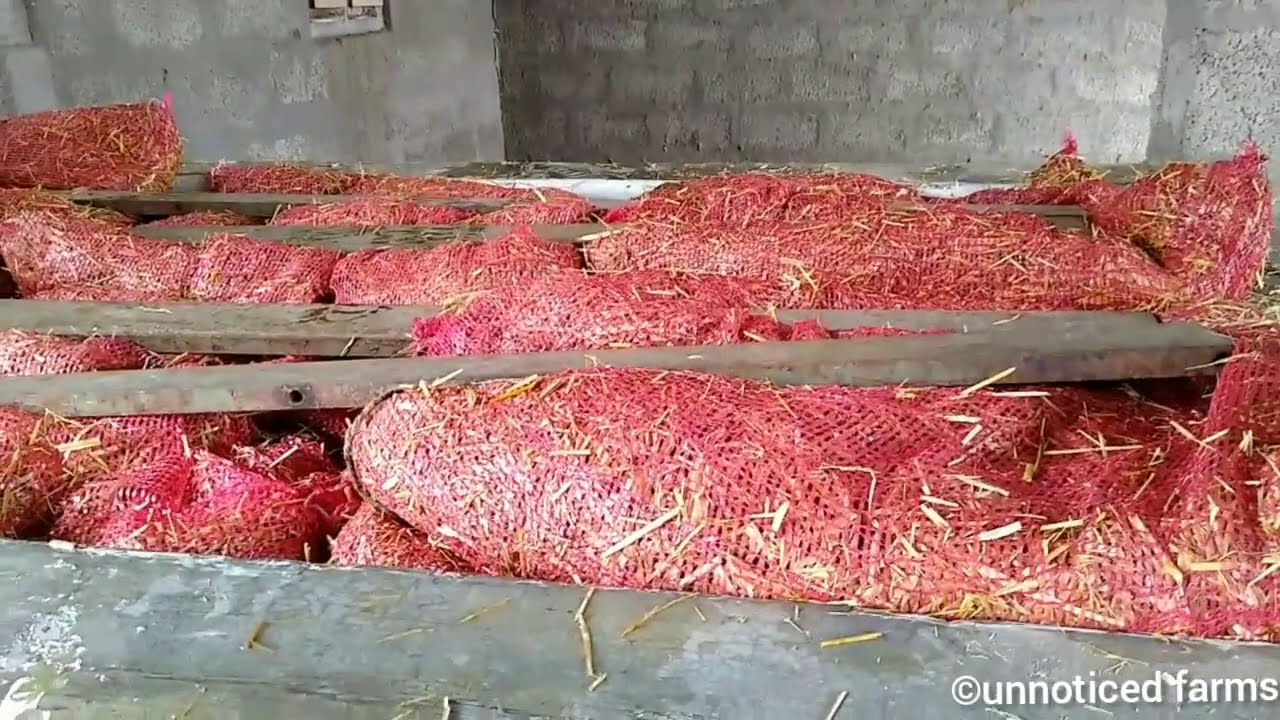The photograph, illuminated naturally, showcases the interior of a stone building with gray brick walls and visible cement. The focal point is a partially-open wooden crate on a wooden floor, filled with bales of hay or straw, wrapped in red mesh packaging with some straw poking through. Near the lower right corner of the image, a white copyright symbol with a 'C' encircled, followed by "UNNOTICED FARMS" in lowercase letters, is conspicuously displayed. The crate, which is covered with old gray wooden beams, takes up much of the image, with multiple bales stacked centrally. The detailed texture of the bricks and wooden elements adds a rustic ambience to the scene.